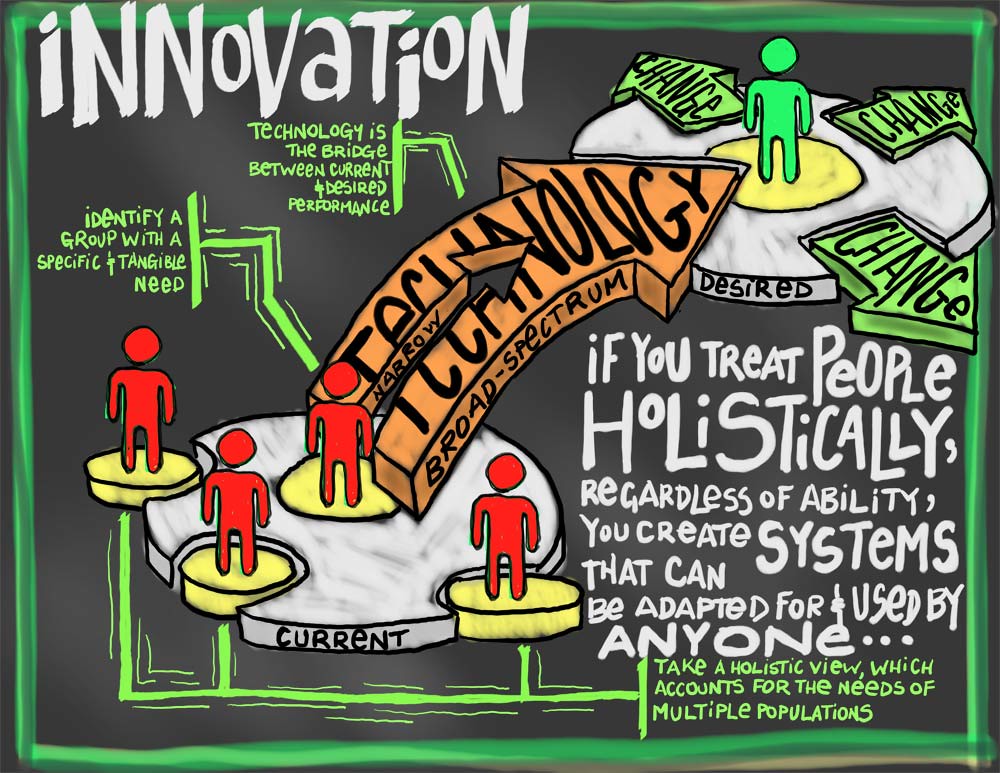The image is a detailed and colorful infographic set against a black background, focusing on the theme of innovation. In the upper left corner, bold white text spells out "Innovation." Centrally, it features two white discs: the lower left disc, labelled "Current," contains four red figures resembling bathroom male icons. The upper right disc, labelled "Desired," has a single green male figure with arrows extending outwards in different directions, marked as "Change." Connecting these two discs is an orange arrow inscribed with "Technology, narrow, broad spectrum," symbolizing the transition facilitated by technology. The infographic also includes important annotations, such as "Technology is the bridge between current and desired performance" and "Identify a group with a specific and tangible need." In the bottom right quadrant, white text reads, "If you treat people holistically regardless of ability, you create systems that can be adapted for and used by anyone. Take a holistic view which accounts for the needs of multiple populations." The visual presentation and the detailed text offer a comprehensive view of how innovation and technology can drive change from the current state to a desired future.